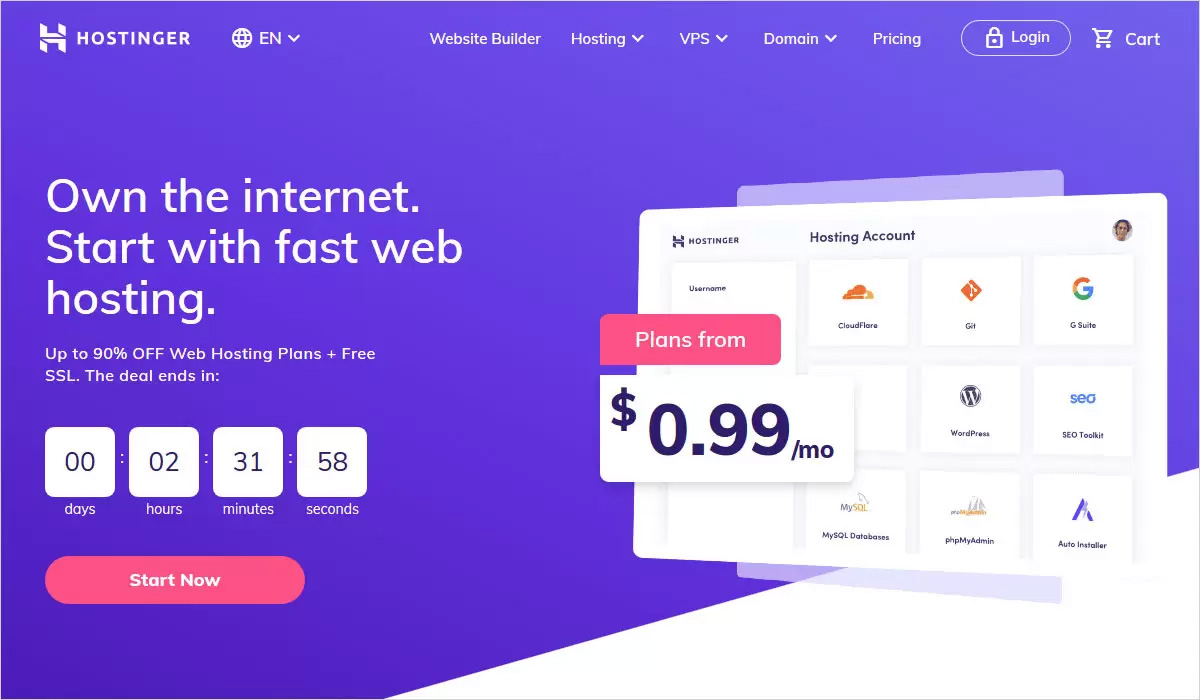On the homepage of Hostinger's website, the design prominently features their branding. The logo, displaying the brand name "Hostinger" in bold letters, is situated on the left side, with a large, stylized "H" that dominates the side, reinforcing their identity. Adjacent to it, a globe icon accompanies "EN" with a dropdown menu, indicating that users can select their preferred language.

The top navigation menu includes several links: "Website Builder," "Hosting" (with a dropdown), "VPS" (also with a dropdown), "Domains" (with a dropdown), "Pricing," and a "Log in" button marked with a lock icon for security. To the far right, there's a cart icon labeled "Cart." The color scheme employs a mixture of purples and blues set against a clean, white background.

The main content area features a compelling call to action on the left side, urging users to "Own the internet. Start with fast web hosting." A promotional offer highlights that web hosting plans are available at up to 90% off, with free SSL included. This limited-time deal is underscored by a countdown timer displaying "Days 00, Hours 02, Minutes 31, Seconds 58," with each unit presented in white boxes with black text.

Below the main text, a striking red button with white text reads "Start Now." To the right, there is a clear indication of pricing: the phrase "Plans from" is written in white text within a purple-blue button-like shape, followed by a white rectangle showcasing the cost of "$0.99/month." This precise and color-coordinated homepage design effectively communicates the key features and offers of Hostinger.